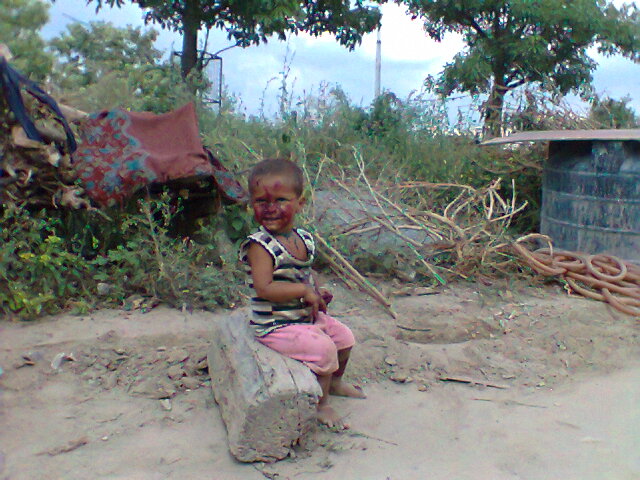This outdoor, daytime photograph captures a child, who appears to be either Hispanic or Black, around 3 years old, sitting barefoot on a cut log situated on a patch of brown soil or dirt. The child wears a black and white striped tank top and pink knee-length pants, and has short hair. Their face is smeared with what appears to be blood, and they look distraught. The background reveals green bushes to the left and some branches with a hose to the right, behind which stands a black barrel with a lid. Further back, there are trees with a red and teal carpet hanging on them, and a possible radio tower under a blue sky with white clouds. The child is placed in a natural setting with shrubs and green foliage around them.